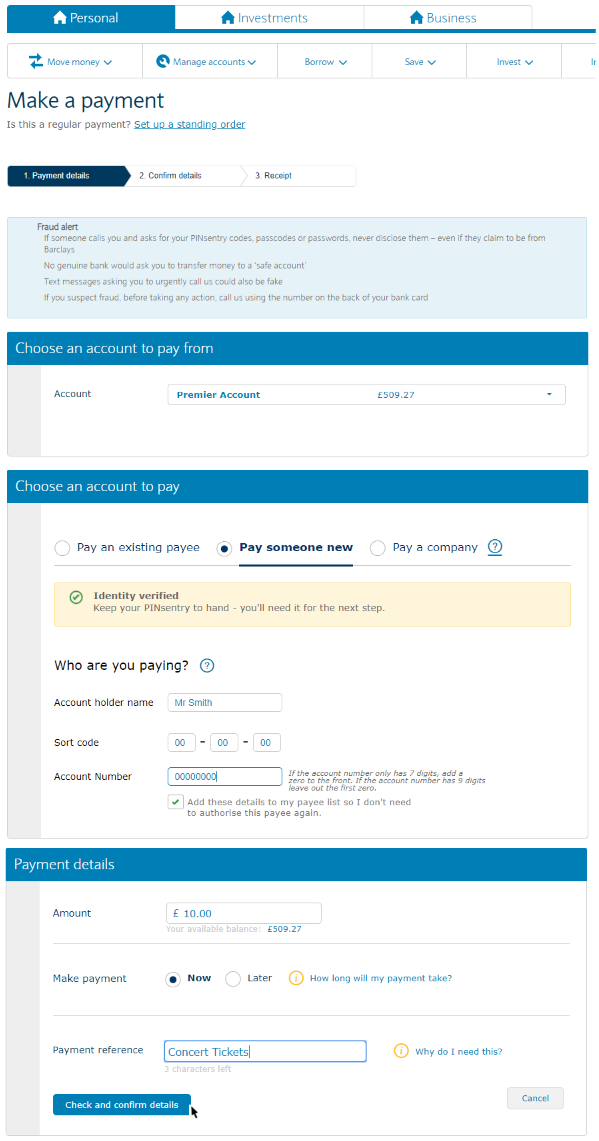The screenshot depicts a payment page on a website with a clean, white background. At the top is a header containing three options. The first option, highlighted with a blue background, white text, and an icon of a house, is labeled "Personal." To its right are two white tabs with blue text and house icons, labeled "Investments" and "Business," respectively.

Below the header are several tabs with white backgrounds and thin gray outlines, featuring blue icons and text. Here are the details of these tabs from left to right:
1. The first tab has arrows pointing right and left, labeled "Move Money," followed by a downward arrow.
2. The second tab shows a blue circle with a white wrench, labeled "Manage Accounts," followed by a downward arrow.
3. Continuing to the right, the subsequent tabs are labeled "Borrow," "Save," and "Invest," each followed by a downward arrow.

Under these tabs, large gray text reads, "Make a Payment." Beneath this header, small gray text asks, "Is this a regular payment?" Next to it, blue underlined text prompts, "Set up a standing order."

Presented below are three tabs indicating the process stages:
1. The first tab, with a dark blue background and white text, reads "1. Payment Details," and features a rightward arrow forming its right side.
2. The second tab, with a white background, reads "2. Confirm Details" and mirrors the design of the first.
3. The third tab, also with a white background, reads "3. Receipt."

At the bottom, a light blue box contains a warning with the title "Fraud Alert" in gray text. Several lines of smaller, light gray text provide critical information advising:
- Never disclose your PIN, Sentry codes, passcodes, or passwords if solicited by someone claiming to be from Barclays.
- No legitimate bank would ask you to transfer money to a "safe account."
- Be cautious of text messages urging urgent callbacks as they may be fraudulent.
- If you suspect fraud, contact the bank using the number on the back of your bank card prior to taking any action.